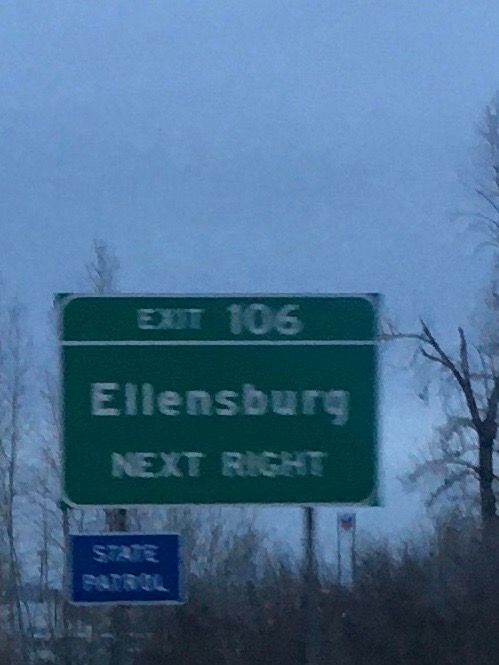This photo captures a foggy and somewhat indistinct scene, possibly due to camera motion, incorrect settings, or heavy air pollution. The sky exhibits a light to medium blue hue, tainted by a pervasive gray haze. The sun is obscured, contributing to the overall murkiness. In the foreground, a group of deciduous trees stands with bare branches, accompanied by brushy undergrowth consisting mostly of barren sticks. To the bottom far left, there is an indistinct structure, possibly a building, though it isn't clearly visible.

Dominating the center of the image is a large rectangular road sign with a green background and white text. This sign reads "Exit 106 Ellensburg Next Right." Below it and to the left is a smaller sign with a blue background and white lettering that indicates "State Patrol."